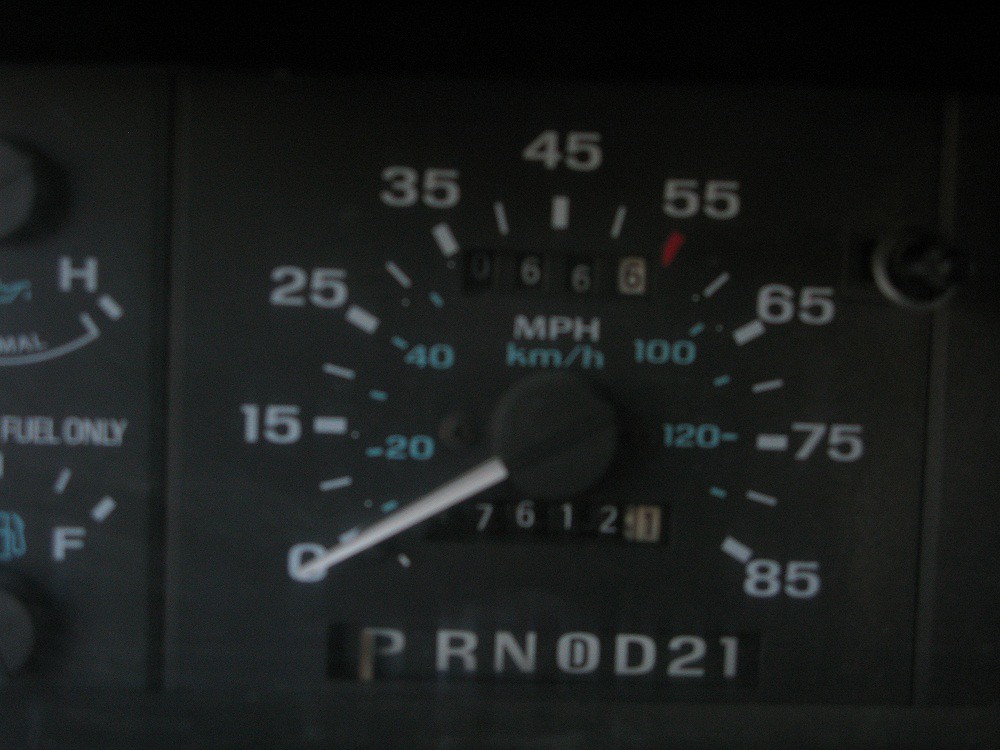The image depicts a partial view of a car dashboard in a black-to-gray gradient. On the left-hand side, there is an indistinguishable blue element next to a control knob, followed by an unreadable blurred line and letters. Just below, there is an "H" with a small dash to the right and slightly underneath it, along with the words "Fuel Only." Adjacent to this text is a partial gas tank symbol above a thick dash line marked with "F" signifying full fuel.

To the right of this section, a detailed speedometer is visible. The speedometer features white numbers and dashes around its circumference, where thicker dashes mark the numbers, and thinner dashes fill the spaces in between. A notable red dash highlights the 55 mph mark. Below the speedometer, the label "MPH" is displayed, and there is an odometer showing the reading "0666," where the first three digits are white on black and the final digit is black on white. The speedometer also has "MPH" written in white and "KM-H" in blue, with corresponding blue numbers around it.

Additionally, beneath the MPH display lies another counter, starting with an unreadable number followed by "612" in white-against-black, and a solitary "1" in black-against-white. Below this counter is a darker rectangular section containing the gear shift indicator. The indicator reads "PRND2L," where the "D" symbol is enclosed within a square with rounded corners, and another "D," "2," and "1" are noted sequentially.